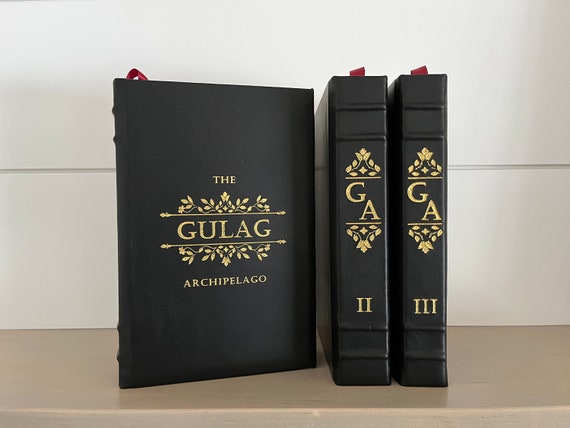This image depicts three black, leather-bound volumes of "The Gulag Archipelago," authored by Aleksandr Solzhenitsyn. The books are positioned upright on a light brown shelf against a white background. Each book features gold lettering and intricate decorations on the cover. The first volume prominently displays "The Gulag Archipelago" with gold embellishments, while volumes 2 and 3 show their spines, marked with the letters "G.A." and Roman numerals II and III, respectively. Red ribbon bookmarks are visible at the tops of all three books, adding a touch of elegance to the set. The background is characterized by gray paneling with distinct lines between each panel, highlighting the neat and orderly placement of the volumes.